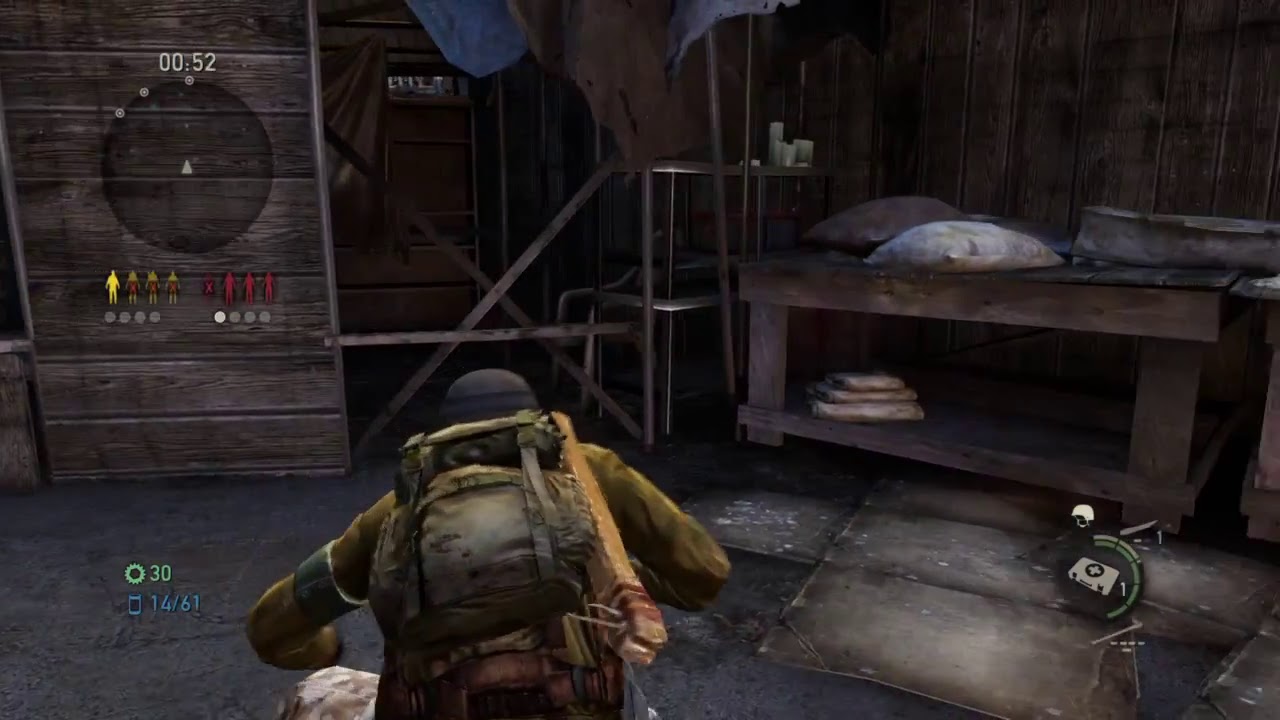The image is a detailed screenshot from a third-person shooter video game, depicting a soldier in a likely abandoned, indoor environment suggestive of a bunker or a warehouse. The scene is animated, revealing the character—a man seen from the back—wearing military-style attire including a black helmet, a green coat, and a matching camo backpack. Strapped to the back of the backpack is a wooden structure, though its purpose is unclear. 

The setting comprises wooden floors and walls with a distinctly worn and filthy look, hinting at the place's abandonment and perhaps cold conditions. There is a makeshift wood table or bench, scattered pillows suggesting it might have served as a bed, a first aid kit on the floor, and folded blankets tucked underneath. Other elements include metal and steel poles, scaffolding to the front, a wooden wall with boards, a visible corner of a window, and various objects like stacks of packages and bags. 

On the game's interface, gauges and indicators present information such as remaining lives, gears, a cell phone count of 14 out of 61, and a med kit icon with a cross symbol and the number 'one,' hinting at the player’s health status. The detailed environment and character design contribute to the immersive, possibly survival-themed gameplay experience.